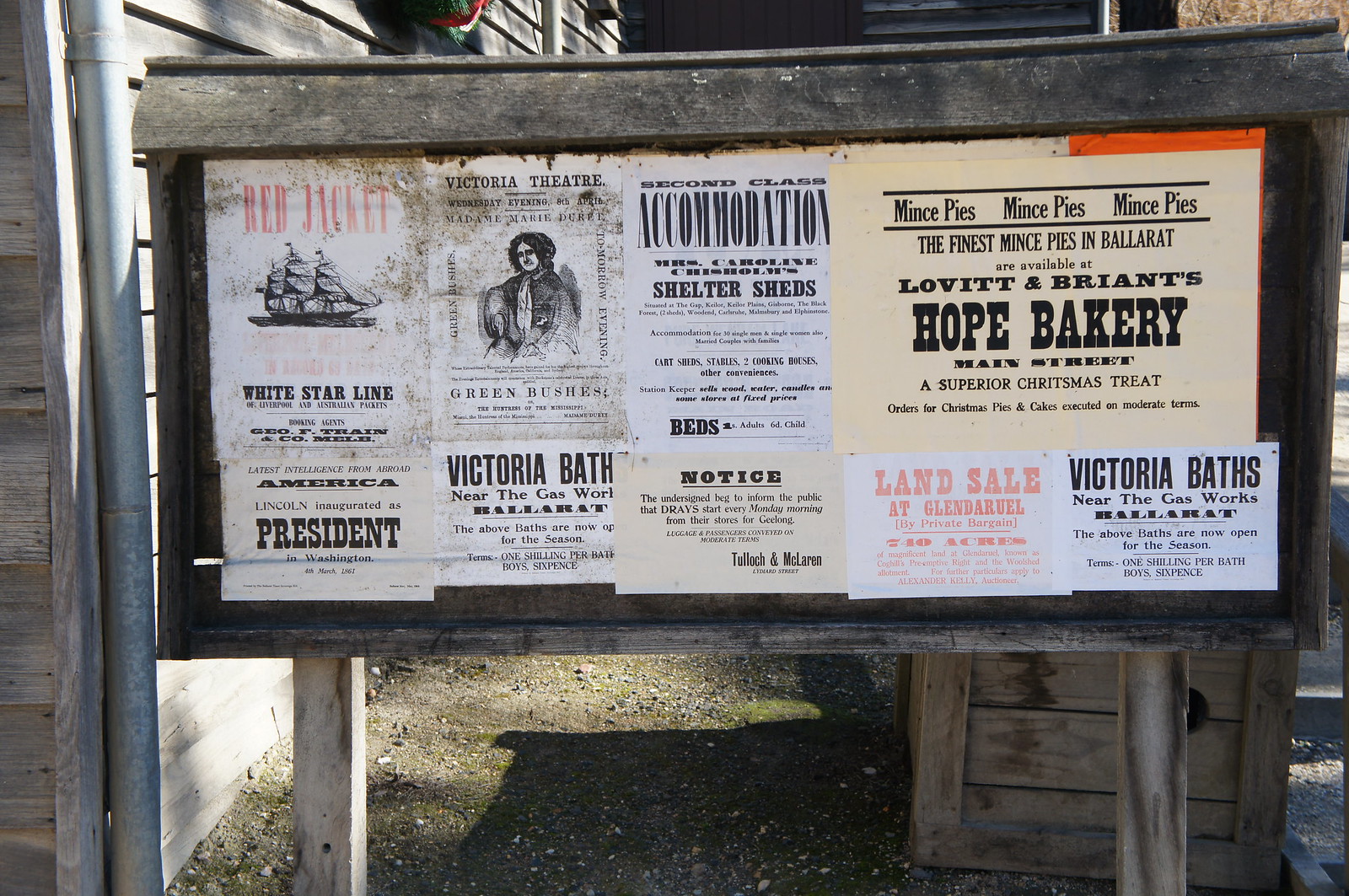The image is a detailed photograph of a weathered, wooden notice board set in a Western-style themed area, possibly a historic reenactment site or movie set, suggesting a location in Ballarat. The board is dark wood and supported by two wooden posts, standing outdoors on a ground of brown soil and rock. Attached to the board are four full-size and five half-size pieces of neutral-colored paper, predominantly yellows and whites, with black text. Among the various notices, one advertises "Levit and Bryant's Hope Bakery" offering "the finest mince pies in Ballarat," another reads "Red Jacket" with a drawing of a boat, and yet another promotes the "Victoria Theatre" with an illustration of a woman. Other papers mention "Second Class Accommodation," "Victoria Baths," "America President," and a "Land Sale at Glendarelle," showcasing a mix of advertisements and public notices consistent with the historical Western theme. The overall scene is enriched by a backdrop of wooden structures and a dusty brown aggregate ground, enhancing the authentic period atmosphere.